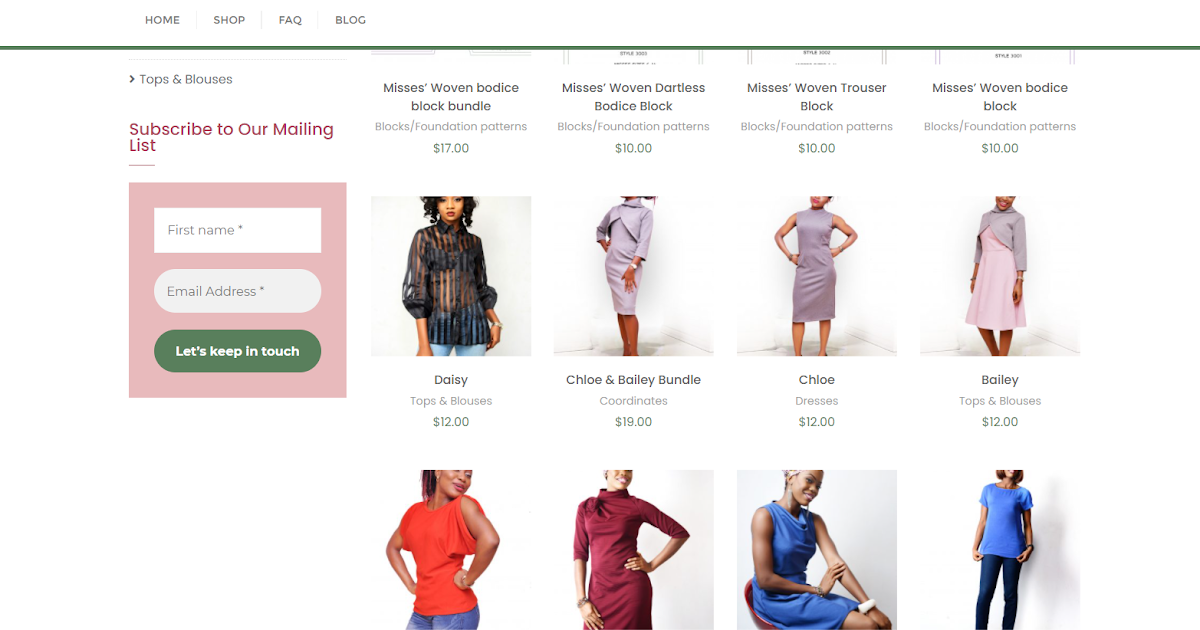A screenshot of a clothing retail website displaying several product thumbnails. In the top-left corner, the navigation menu features tabs labeled "Home," "Shop," "FAQ," and "Blog," separated by a green line. Below the menu, a section titled "Tops and Blouses" showcases four main product categories:

1. **Mrs. Woven Bodice Block Bundle**: Listed under "Blocks / Foundation Patterns," priced at $17.
2. **Mrs. Woven Dartless Bodice Block**: Priced at $10.
3. **Mrs. Woven Trouser Block**: Priced at $10.
4. **Mrs. Woven Bodice Block**: Priced at $10.

Each product displays a thumbnail of a woman modeling the respective clothing item. Below this row, another row highlights:

1. **Daisy Tops and Blouses**: Priced at $12, modeled by a woman wearing a slightly see-through black top.
2. **Chloe and Bailey Bundle Coordinates**: Priced at $12, showcased by a woman in a purplish dress.
3. **Chloe Dresses**: Priced at $12, illustrated by another purplish dress.
4. **Bailey Tops and Blouses**: Priced at $12, accompanied by an image of a woman in a pink dress with a purplish cardigan.

At the bottom of the page, there are additional images of women in a variety of outfits, including a red shirt, a red dress, a blue dress, and a blue shirt.